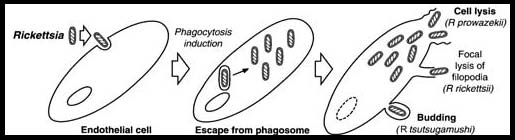The image is a detailed scientific diagram, primarily in black and white, with a black border surrounding the entire rectangular frame. The background is white, creating a stark contrast for the labeled elements. The focus of the diagram is on the lifecycle of Rickettsia within an endothelial cell. The sequence of processes depicted involves several stages: phagocytosis induction, escape from the phagosome, cell lysis, focal lysis of philopodia, and budding. The diagram includes labeled stages with accompanying illustrations, such as arrows indicating the direction of the processes. Notably, it mentions different types of Rickettsia, specifically R. prowazekii, R. rickettsii, and R. tsutsugamushi. The stages are clearly outlined with respective descriptions and visuals, making it a comprehensive depiction likely intended for educational use in a scientific setting, such as a chemistry or biology classroom. The diagram's elements span the entire image, leaving no room for any extraneous details.